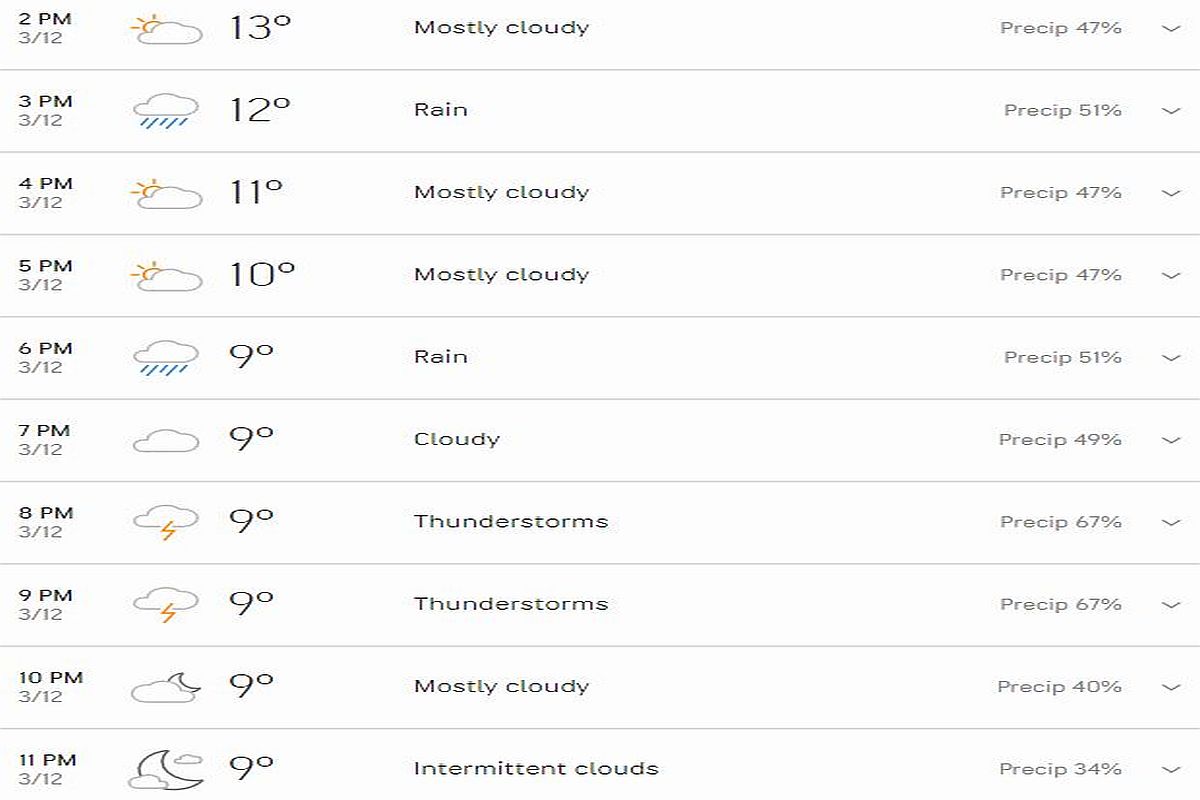A screenshot of a weather forecast webpage captures hourly predictions for March 12th, starting at 2 p.m. and ending at 11 p.m. The layout is borderless and features a series of rows, each indicating the weather conditions for a specific time. At 2 p.m., the weather is partly cloudy with a high of 13°C and a 47% chance of precipitation. By 3 p.m., conditions shift to rain with a temperature of 12°C and a 51% precipitation probability. At 4 p.m., it is mostly cloudy with intermittent sunshine and a temperature of 11°C, with precipitation holding steady at 47%. This mostly cloudy pattern, accompanied by sun, continues at 5 p.m., while the temperature drops to 10°C and precipitation remains at 47%. By 6 p.m., rain returns, forecasting a temperature of 9°C and a 51% chance of rain. The weather prediction continues in a similar format until 11 p.m., where the forecast shows intermittent clouds with a temperature holding at 9°C and a reduced precipitation chance of 34%, depicted by a moon partially obscured by clouds.